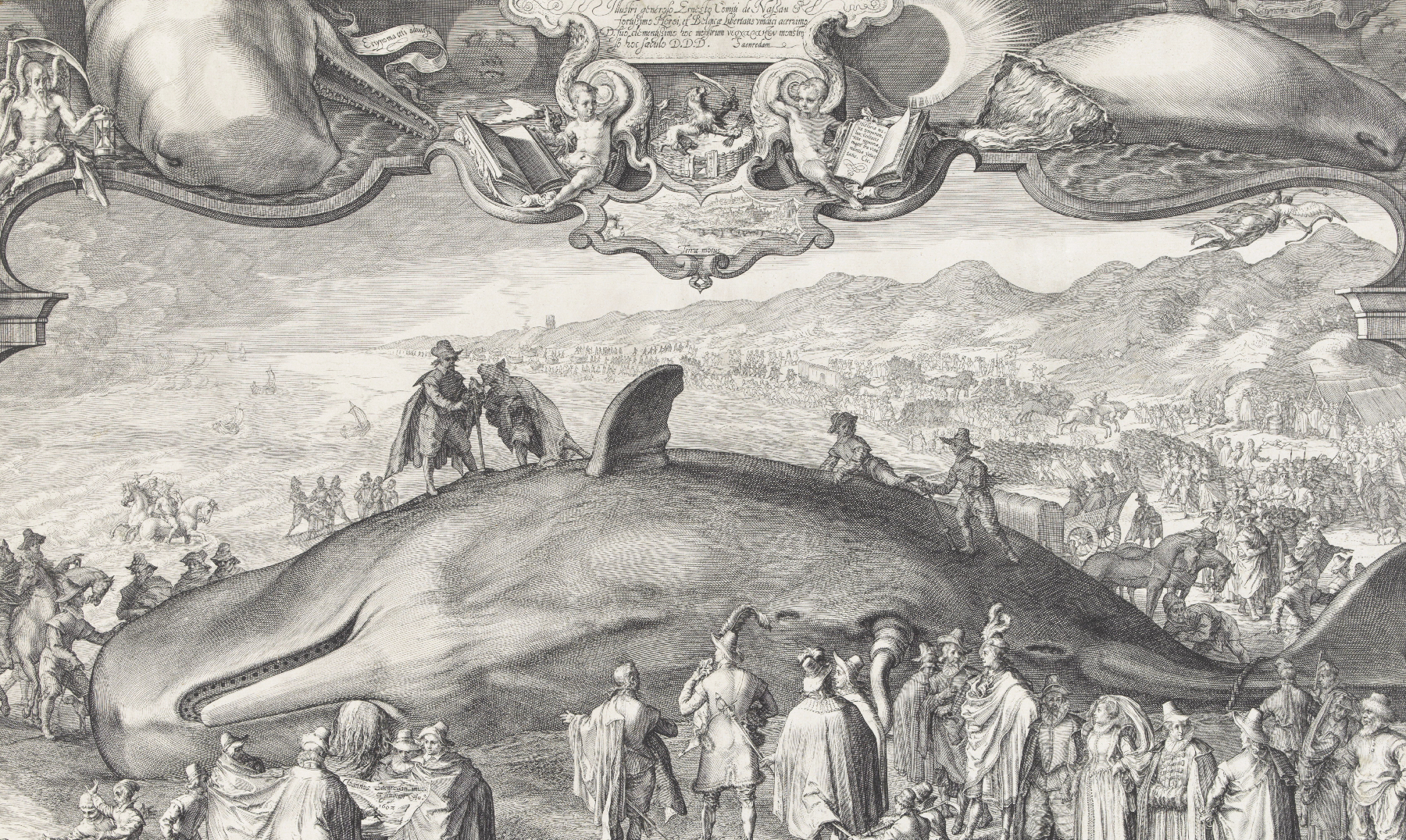This is a very old, intricate black and white pencil drawing, depicting a large sperm whale that appears to be beached or lying on the ground on its side, with its belly facing the viewer and its fin up in the air. The scene is bustling with activity as a significant number of people, many of whom are dressed in regal attire, gather around the enormous creature. A few individuals, including a man in a cape, top hat, and holding a cane, stand on top of the whale. In the background, a mountainous landscape is visible, populated with even more onlookers and a couple of horses. 

The top portion of the artwork features a curved border adorned with two cupids on each side and two smaller sperm whales, adding to the ornate design. There are also depictions of naked men, children, sad moon faces, and various animals, contributing to the scene's complexity. The upper border includes a plaque with writing, possibly a signature, though it's not legible. This detailed drawing appears to be from an old textbook, capturing an illustrative moment where people might be examining the whale for potential food or out of sheer curiosity.